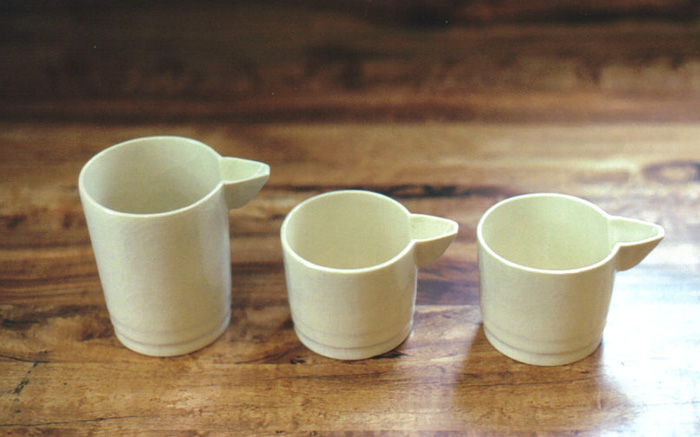The image showcases three ivory-colored measuring cups arranged in a row on a tan light brown wooden table with a shiny, reflective surface. The taller cup is positioned at the back, while the two smaller, identical cups are in the front. Each cup features a spout on the right-hand side and three ring indentations around their bases, adding texture. The wood grain of the table is visible, contrasting with the lighter color of the cups. Light from the right side of the frame creates a bright glare on the table, making that area difficult to see clearly. The upper part of the image is darker and blurred, drawing focus to the cups. The photo, taken indoors, emphasizes the clean simplicity and arranged alignment of the cups, which appear empty.